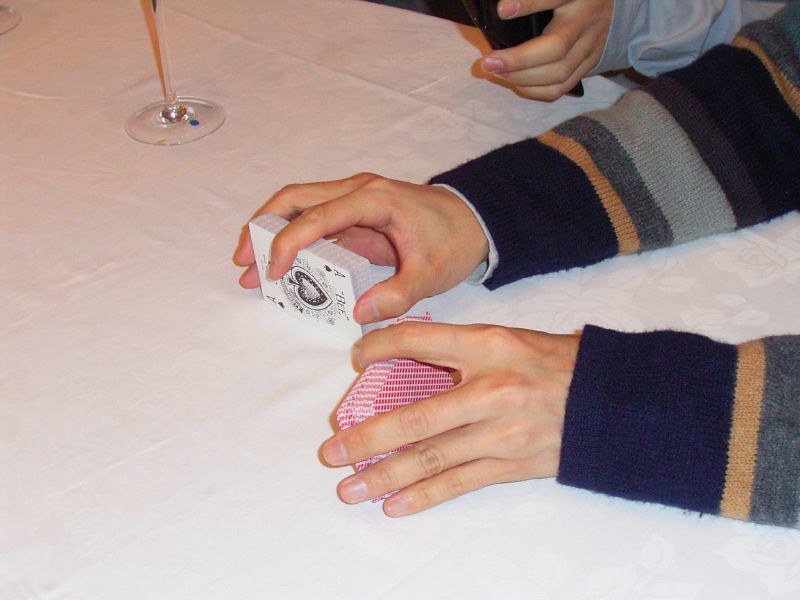A detailed photograph captures a tabletop covered with a slightly wrinkled white tablecloth, still showing fold creases. The central focus of the image is on two hands and forearms clad in a striped sweater of blue, gray, and beige hues, holding a deck of cards in the midst of being shuffled. The stem and base of what appears to be either a champagne flute or a vase are partially visible on the table, its top obscured from view. Beside the dealer, another hand belonging to a person in a light blue shirt holds a cell phone. The casual, yet intimate setting suggests a moment of anticipation before a game begins.